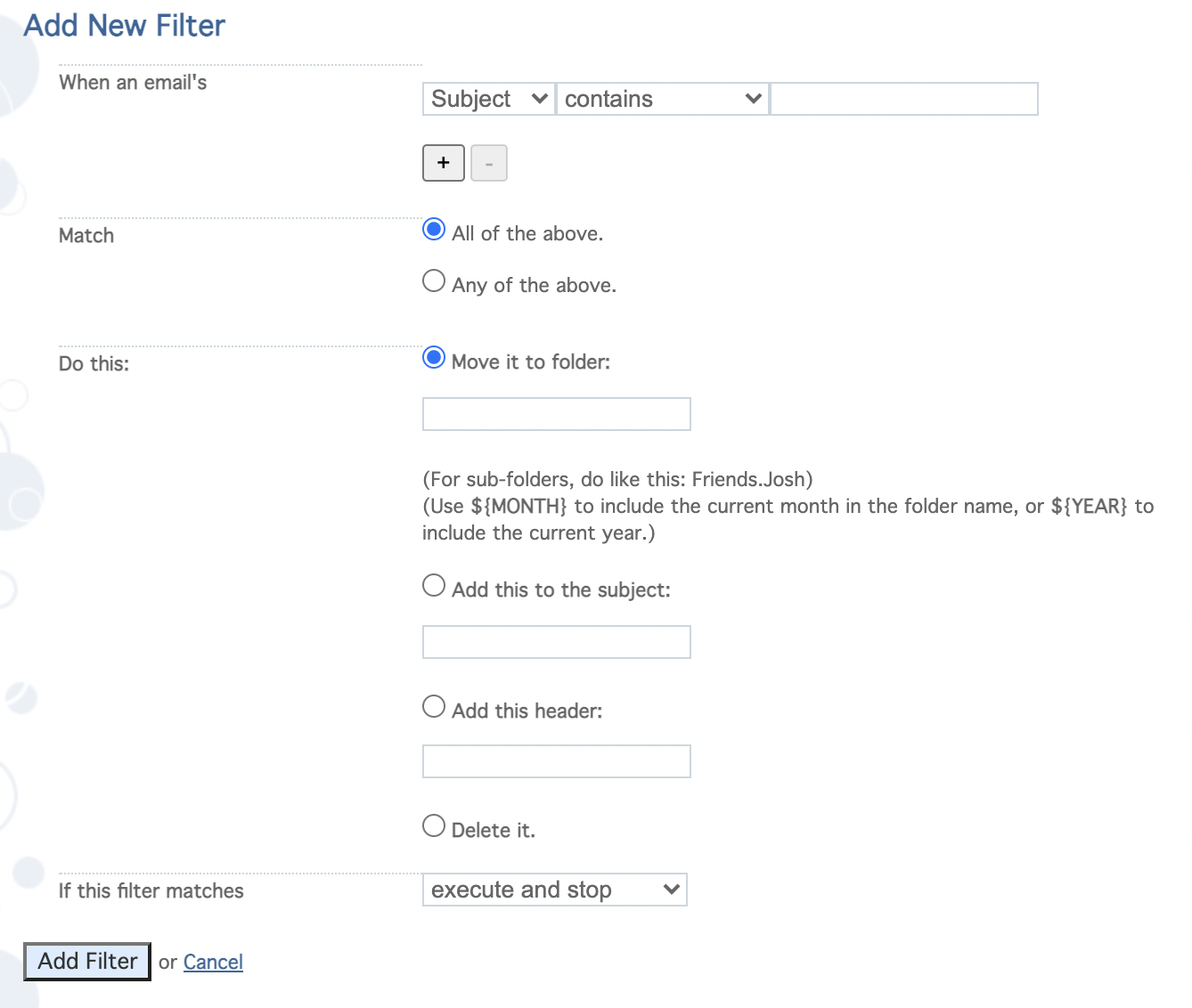A screenshot showcasing the "Add New Filter" page for setting up email filters. At the top left corner, the title "Add New Filter" is highlighted in blue. Below the title, there's an "Email Filter" section.

1. First Filter Condition:
   - On the left, it states "When an email's..."
   - On the right, there are two drop-down boxes:
     - The first drop-down box is labeled "Subject" and the second one "contains".
     - Accompanied by a text field for entering specific subjects.
     - Plus ("+") and minus ("-") buttons are available for adding or removing conditions.

2. Matching Criteria:
   - Below the filter conditions, there's a "Match" section with two radio buttons:
     - "All of the above" (selected)
     - "Any of the above"

3. Filter Actions:
   - The "Do this" section provides options for what to do with matching emails:
     - "Move to folder" is selected, with a text field provided for specifying the folder.

4. Additional Settings:
   - An option labeled "For subfolders do like this" followed by a hint for usage.
   - Additional hints on how to use month and year filters.
   - Options to:
     - Add this to Subject
     - Add this to Header
     - Delete it

5. Execution Criteria:
   - The section "If this filter matches" with another drop-down box.
   - The options "Execute" and "Stop" are selected.

6. Bottom Controls:
   - At the bottom left, there are two buttons:
     - A light blue square button labeled "Add Filter"
     - A "Cancel" link styled as a hyperlink.

This detailed layout provides a comprehensive view of how to create and manage email filters on the filter settings page.